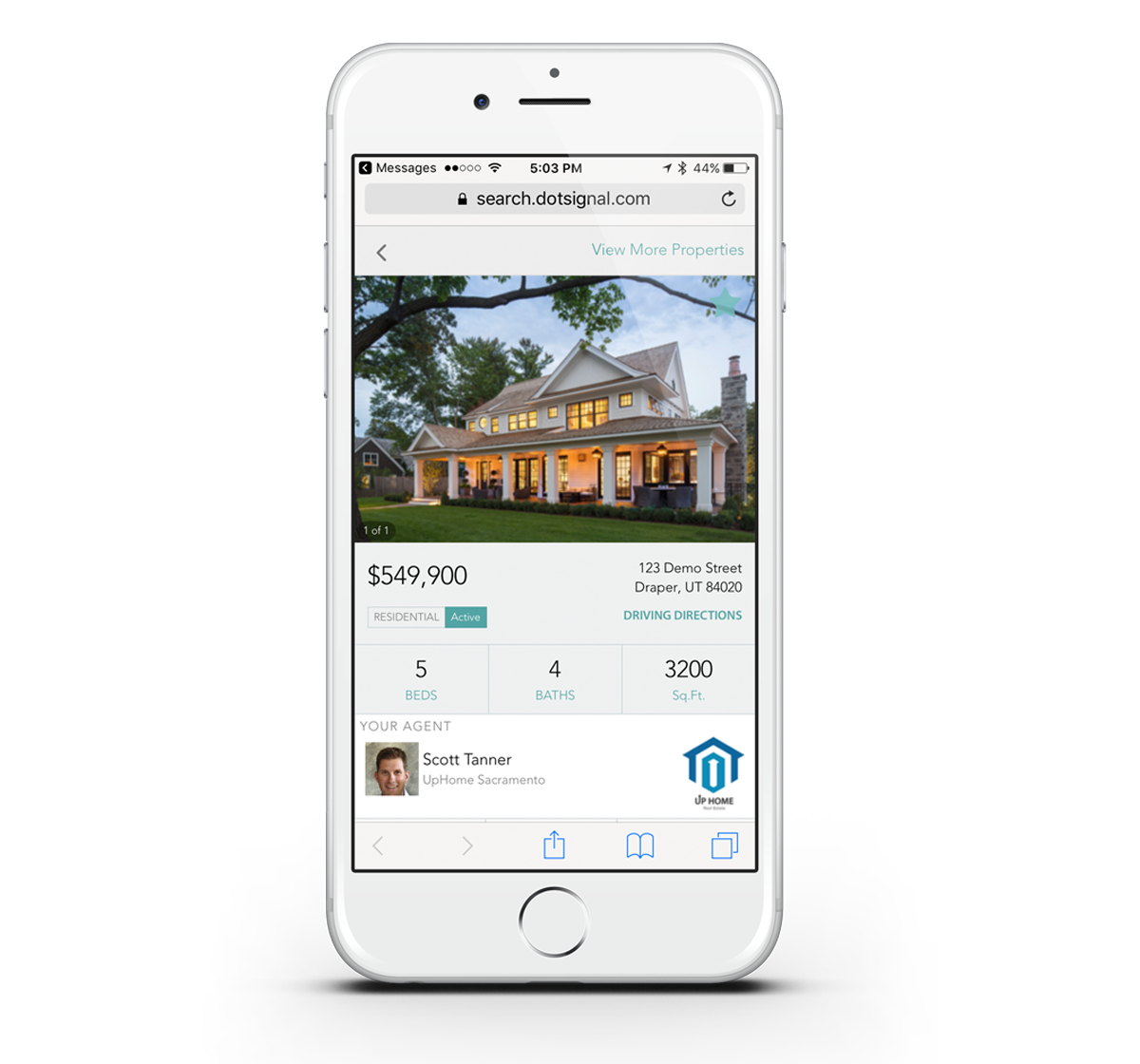This image is a detailed screenshot of a mobile phone, prominently displaying both the device and a real estate webpage. The phone itself is shown with its physical characteristics: three buttons located on the top left edge, likely the volume up and volume down buttons, and a power button on the right edge. The device also features a small front-facing camera at the top and a central button at the bottom.

The webpage being viewed is a real estate listing for a colonial-style house priced at $549,900, located in the fictional address of 123 Demo Street, Daper, Utah, 84020. Below the address, a link for driving directions is available. The property details include five bedrooms, four bathrooms, and an overall area of 3,200 square feet. 

The listing is represented by Scott Tanner from Up Home, Sacramento. His picture and the Up Home logo, which is a blue house, are displayed on the page. Additionally, an address bar at the top of the browser shows a secure connection with a lock symbol and reads "search.signal.com."